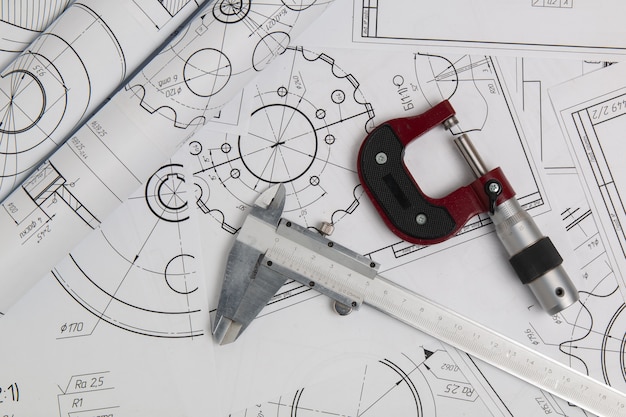The image depicts a drafting board covered with detailed architectural and mechanical drawings, primarily in black and white line illustrations. Central to these illustrations is a detailed depiction of a gear, surrounded by numerous numerical diagrams and measurements crucial for its installation or recreation. The drawings are spread flat on the board, with a few rolled-up sheets visible on the sides. Prominently featured on top of the papers is a long metal ruler and a silver and red tool resembling a spanner or clamp, possibly used for precise adjustments or balancing, notable for its intricate design including a knob and a possibly wooden component on one side. The overall scene is a meticulous arrangement ideal for technical drafting and detailed mechanical design.